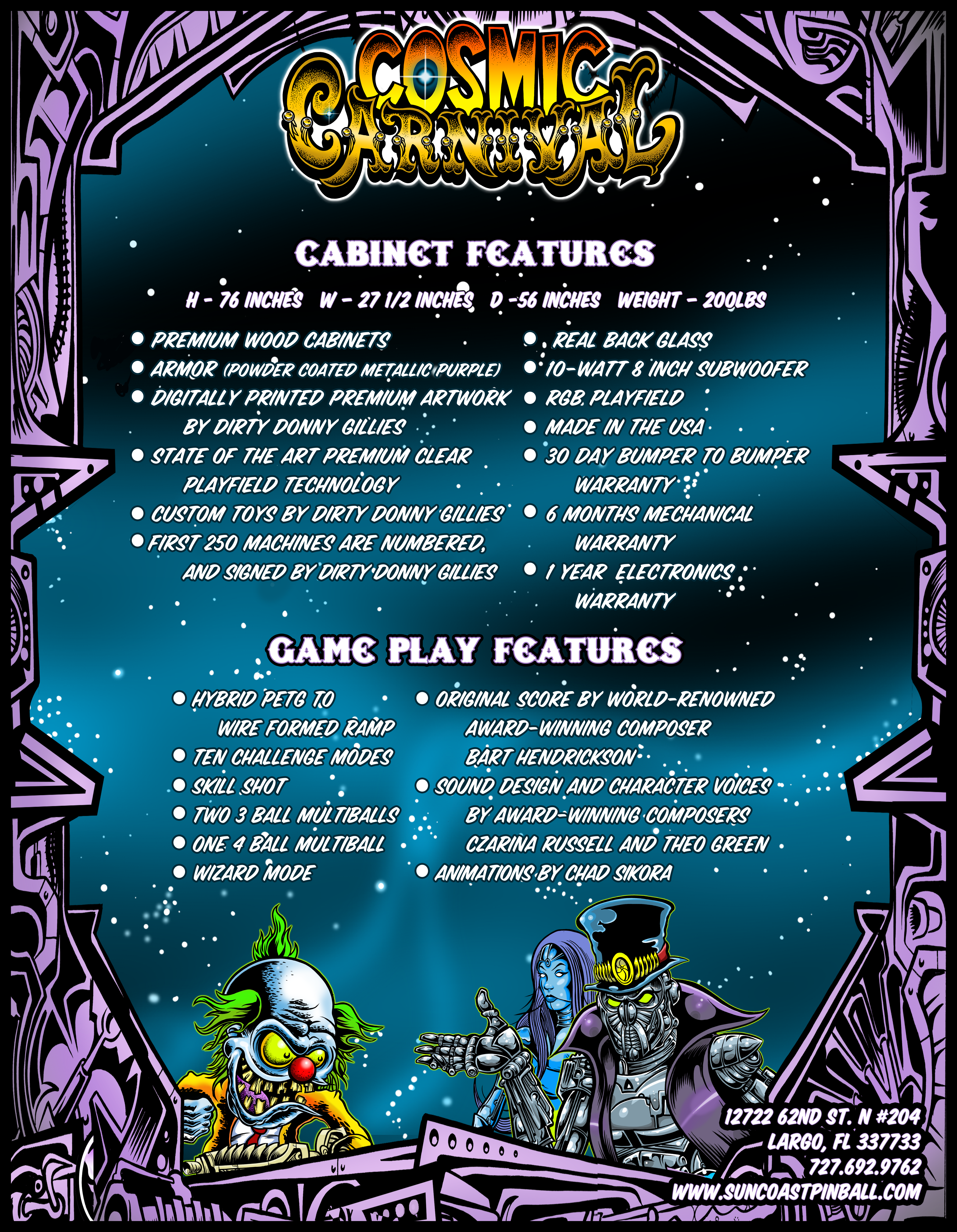This advertisement poster for Suncoast Pinball's "Cosmic Carnival" showcases an engaging and vibrant design. The top of the poster displays "Cosmic Carnival" in striking orange and yellow lettering, set against a backdrop encased by a purple and black border adorned with various geometric shapes. Below, a vivid array of cartoon characters captures attention: an evil clown with green tufts of hair on the lower left, and a menacing monster robot in a black top hat accompanied by a blue-skinned woman with a purple headscarf on the lower right. At the center of the poster, detailed specifications for a pinball machine cabinet are provided: height of 76 inches, width of 27.5 inches, and depth of 56 inches. The cabinet features premium wood construction, backlit by real black glass, and includes digital premium artwork and custom toys, with the first 250 machines being numbered and signed. The gameplay features are equally impressive, boasting an original score by an award-winning composer, animations by Chad Sikora, Wizard Mode, 10 Challenge Mode skill shots, and multiple ball options. The machine comes with a 30-day warranty, a six-month mechanical warranty, and a one-year electronics warranty. Contact details for the company are also displayed: located at 12722 62nd Street North, Suite 204, Largo, Florida 33773, with additional reach via www.suncoastpinball.com and phone number 727-692-9762.